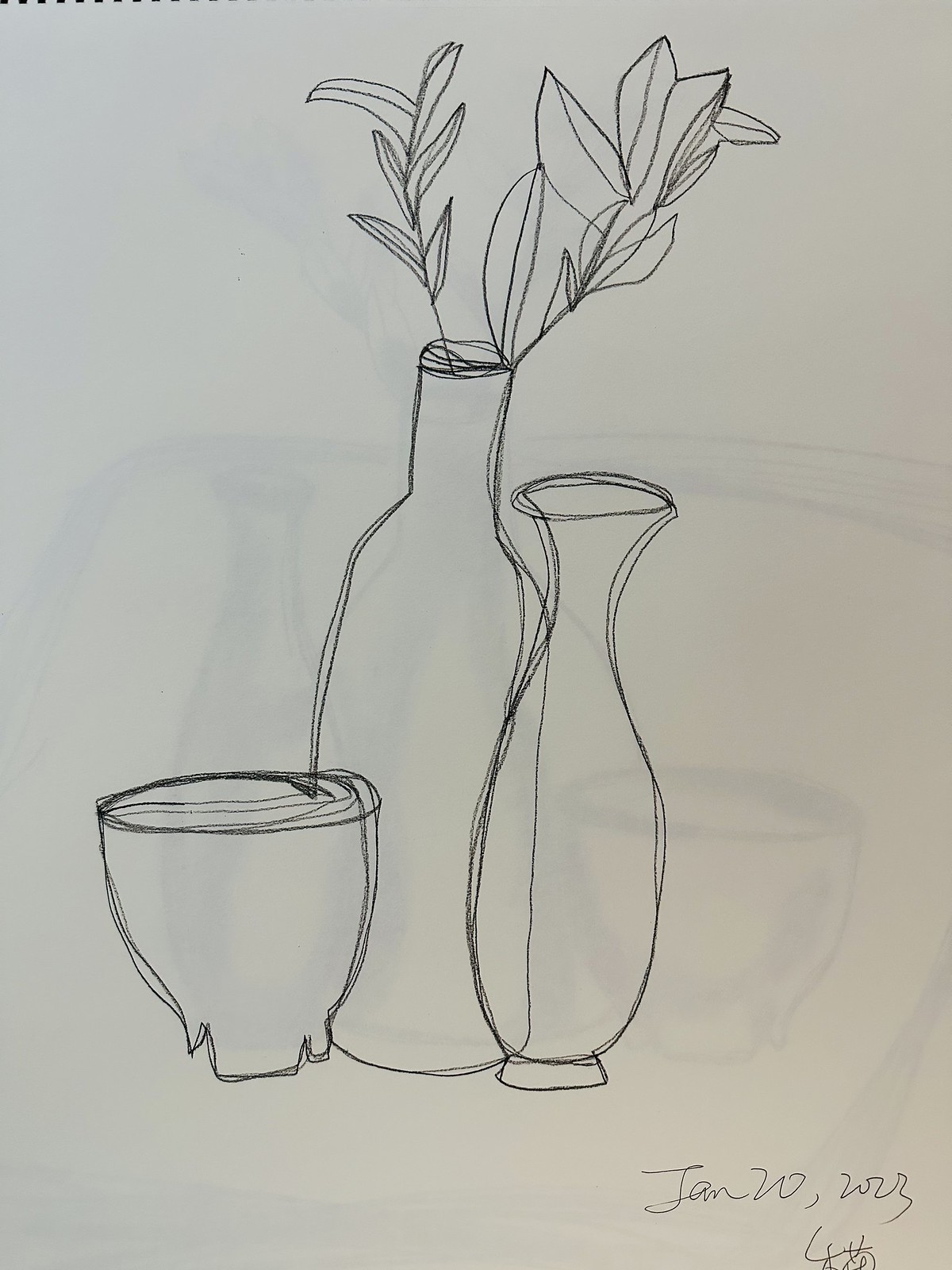A finely detailed pen sketch captures a serene still life arrangement composed of three distinct objects. To the right, a beautifully rendered vase with a curvaceous, narrowing body reminiscent of a pilsner glass stands prominently, its base clearly defined. To its left, a taller bottle with an elegant, slimmer neck supports several stems and leaves sprouting from its opening, adding a touch of organic life to the composition. Further left, there is a small container that could either be a glass or an unused plant pot, minimalist in design yet rich in potential. The artist has meticulously gone over the lines multiple times, creating nuanced highlights and giving the drawing depth and texture. The sketch appears to be executed with either a very fine pen or a sharp graphite pencil on a light gray background. In the bottom right corner, the artist’s signature, dated January 20th, 2023, is accompanied by what seems to be Japanese characters, adding a personal and cultural touch to the artwork.